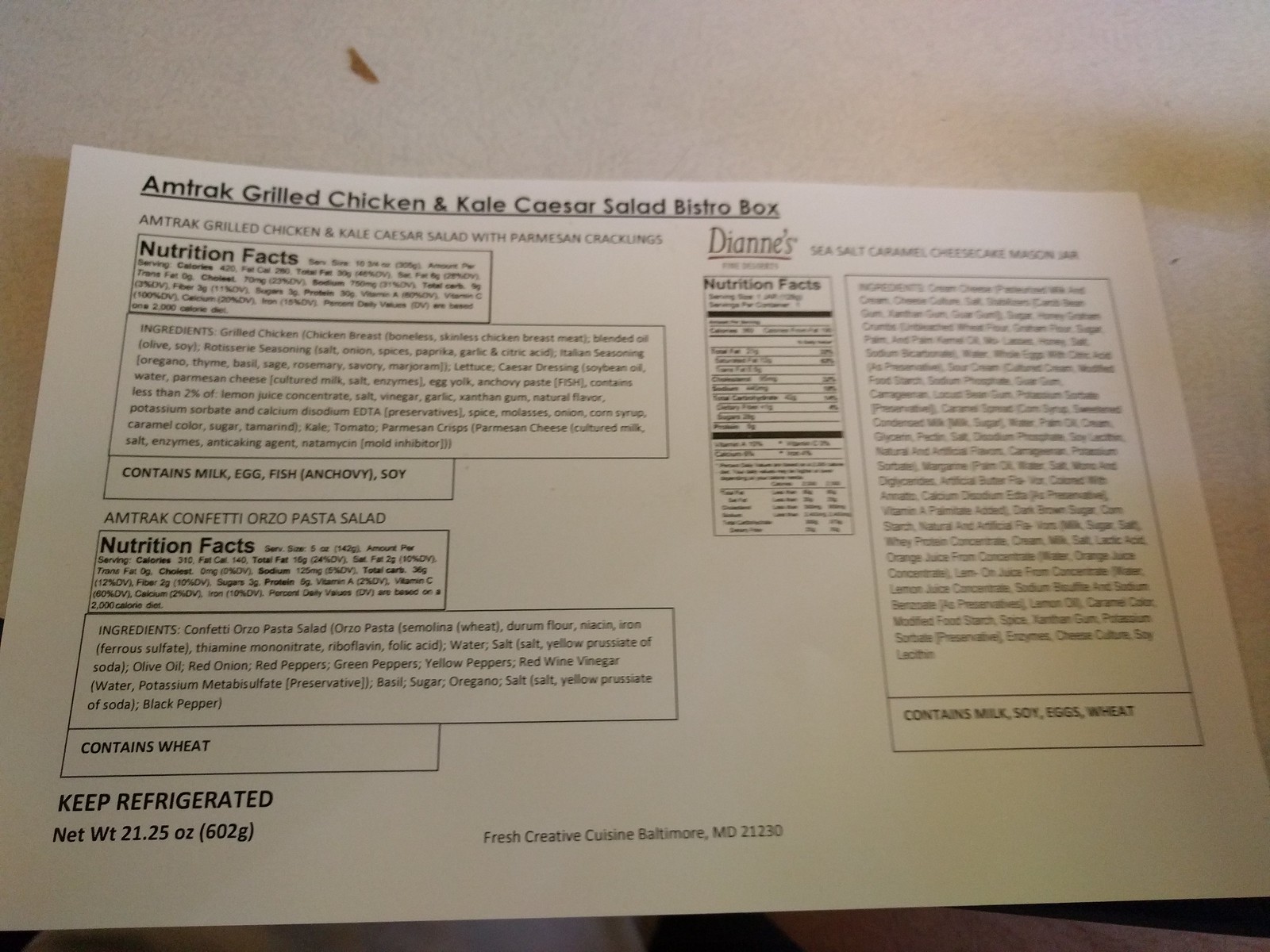The image depicts a white sheet of paper laid out on a white table, with detailed nutritional information likely printed from packaging. At the top of the paper, the title reads "Amtrak Grilled Chicken and Kale Caesar Salad Bistro Box" in black type. This section includes nutrition facts and an ingredients list, which indicates the salad contains milk, egg, fish (anchovy), and soy. Below, it mentions "Amtrak Confetti Orzo Pasta Salad" along with its nutrition facts and ingredients, noting it contains wheat. At the bottom of the paper, it specifies "Keep Refrigerated," lists the net weight as 21.25 ounces (602 grams), and provides the source as "Fresh Creative Cuisine, Baltimore, Maryland, 21230." On the side of the page, another section highlights "Diane's Sea Salt Caramel Cheesecake Mason Jar," accompanied by its own nutrition facts and ingredients. It emphasizes that the cheesecake contains milk, soy, eggs, and wheat. The image seems to be in black and white, with the paper sitting on a white desk, and a small piece of brown paper at the top.